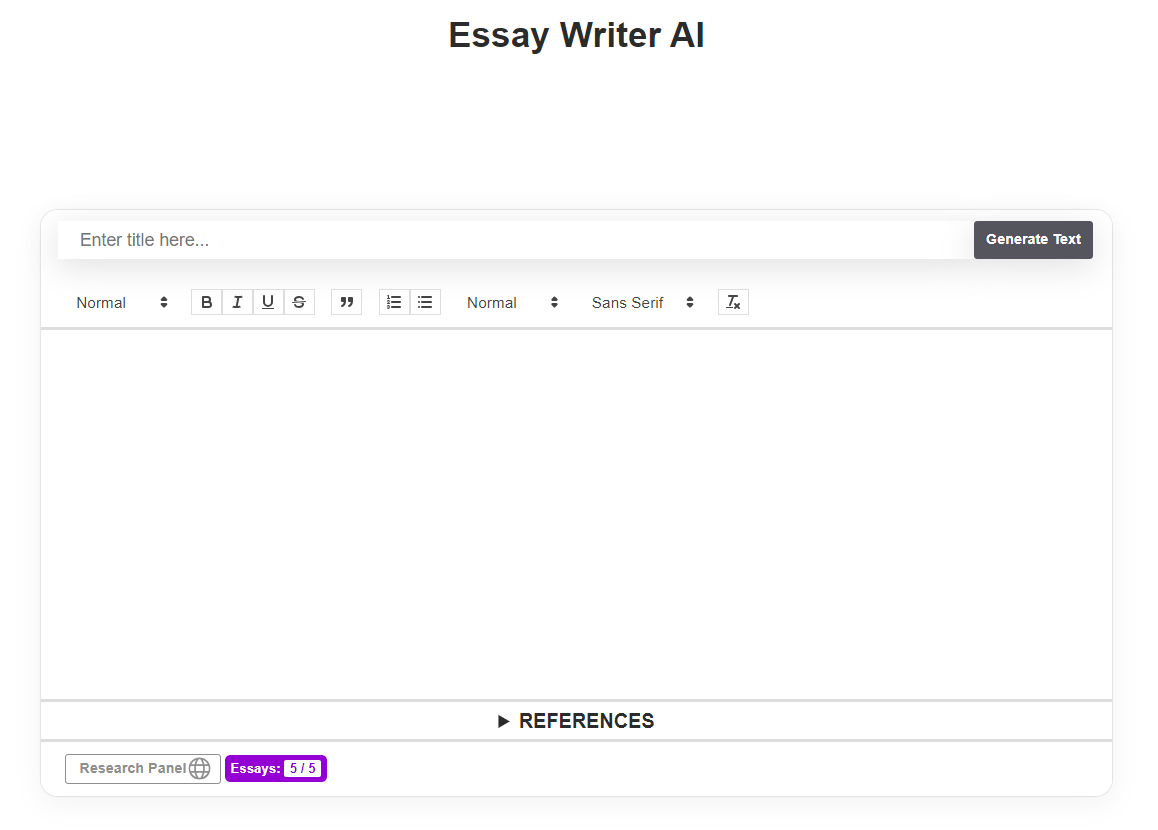The website depicted is Essay Writer AI, characterized by a minimalist and user-friendly interface.

The homepage is dominated by a clean, bright white background. Centrally positioned at the top, the page features a prompt reading "Enter Title Here." Adjacent to this prompt, a prominent black box labeled "Generate Text" invites user interaction. Beneath these elements, options for text styling are available, with the default label 'Normal' visible, accompanied by 'Sans Serif' among other stylistic icons.

In the center of the page, an expansive blank white box serves as the main workspace. Just below this area, a white strip bears the word "References" in bold black letters, paired with a right-pointing arrow, leading users to additional resources. Directly beneath, there is a "Research Panel" which includes a notable label "Essays 515" displayed within a distinct blue box, differing from the otherwise monochromatic theme.

The interface is devoid of company branding, maintaining a stark black-and-white appearance with minimal color accents, notably the blue "Essays 515" box. The solitary page of the site offers a straightforward, uncluttered layout aimed at providing ease of use and focused functionality.